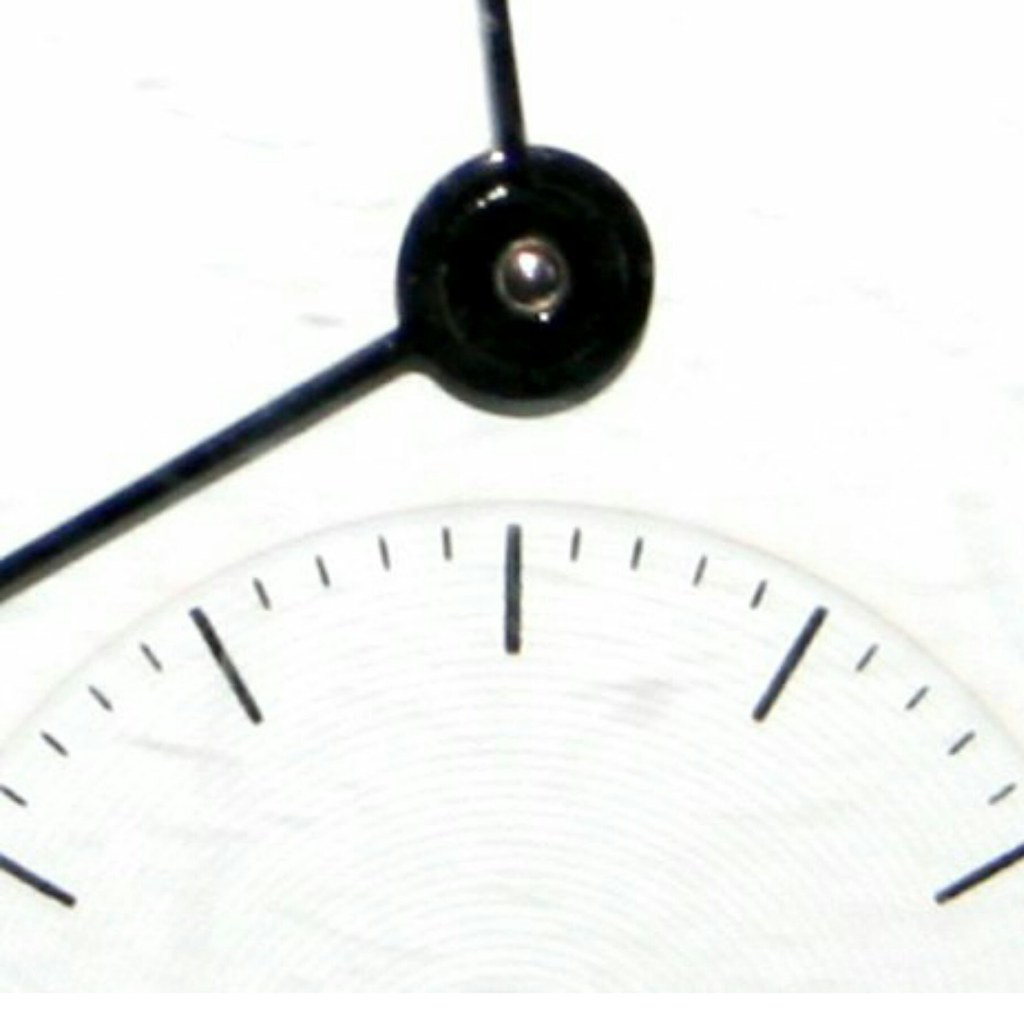The image depicts an extremely close-up view of a clock face, showcasing intricate details. The background is a pristine white. At the center of the image, a black circle serves as the hub from which two black hands extend: one points upwards, and the other angles towards the bottom left. These hands appear to be made of a metallic black material. Nested at the hub is a brown ring encircling a silver element, possibly a bolt. The zoomed-in perspective excludes any numbers on the clock face, leaving only the white surface and the black markings visible. Towards the bottom edge of the image, a partial view of a semicircular ring with black measurement lines indicates the positions where the hour markers (12, 1, 2, 10, 11) and their respective minute divisions would typically be located. The lines extend out of the frame, further emphasizing the close-up nature of the photo.